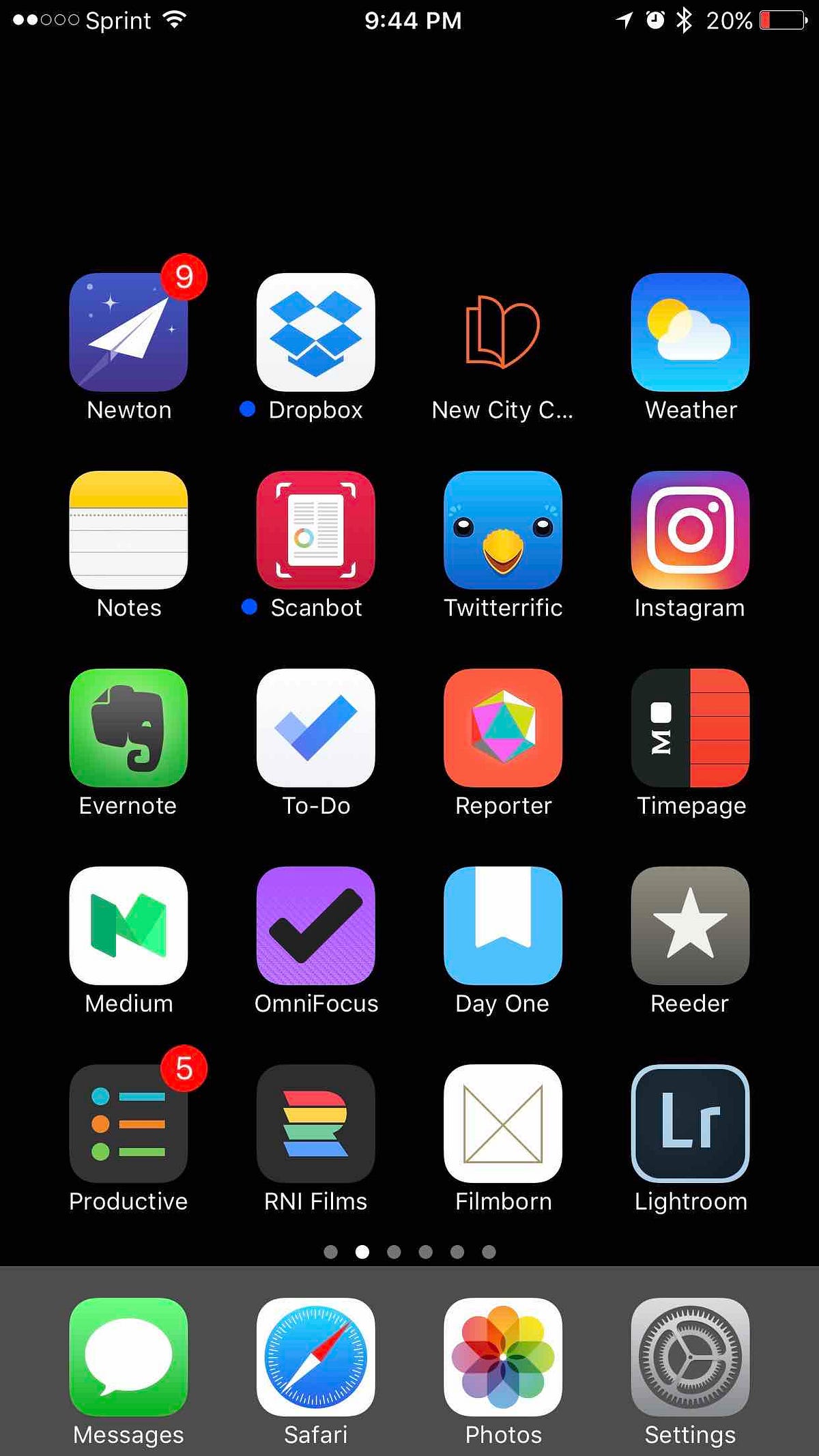The image displays a smartphone screen with various app icons arranged in a grid. 

- The top section shows system information on a black background, including the time displayed as 9:42 PM, a battery level at 10%, and standard signal indicators featuring two white dots and three yellow dots.
- Below this, the first row of icons includes a gray rectangle labeled "Settings" featuring a gear symbol.
- Moving to the right, there is a green square labeled "Messages" and a white square labeled "Safari."
  
Next, we have a collection of distinctly-colored leaves displayed within the "Photos" icon, featuring an orange leaf, a yellow leaf, a green leaf, a blue leaf, and a red leaf against a white background.

- Further to the right, there is a gray square icon with a gear, indicating "Settings," once again.
- The screen then shows a white square for "Dropbox" and a new cityscape icon for a weather app displaying a cloud and yellow sun on a blue background.
- The "Notes" app has a notepad icon with a yellow top.
- The "Scanbot" app is marked by a red square.
- The "Twitter" app features its blue icon with a yellow beak.
- The "Instagram" app is a purple icon, and the "Evernote" app shows a green square.
- Additionally there is a blue checkmark icon, indicating some reporting app.
  
The bottom section includes various other icons and names of likely-used apps noted, such as "Reporter," "Time Page," "Video," and "Stay Productive."